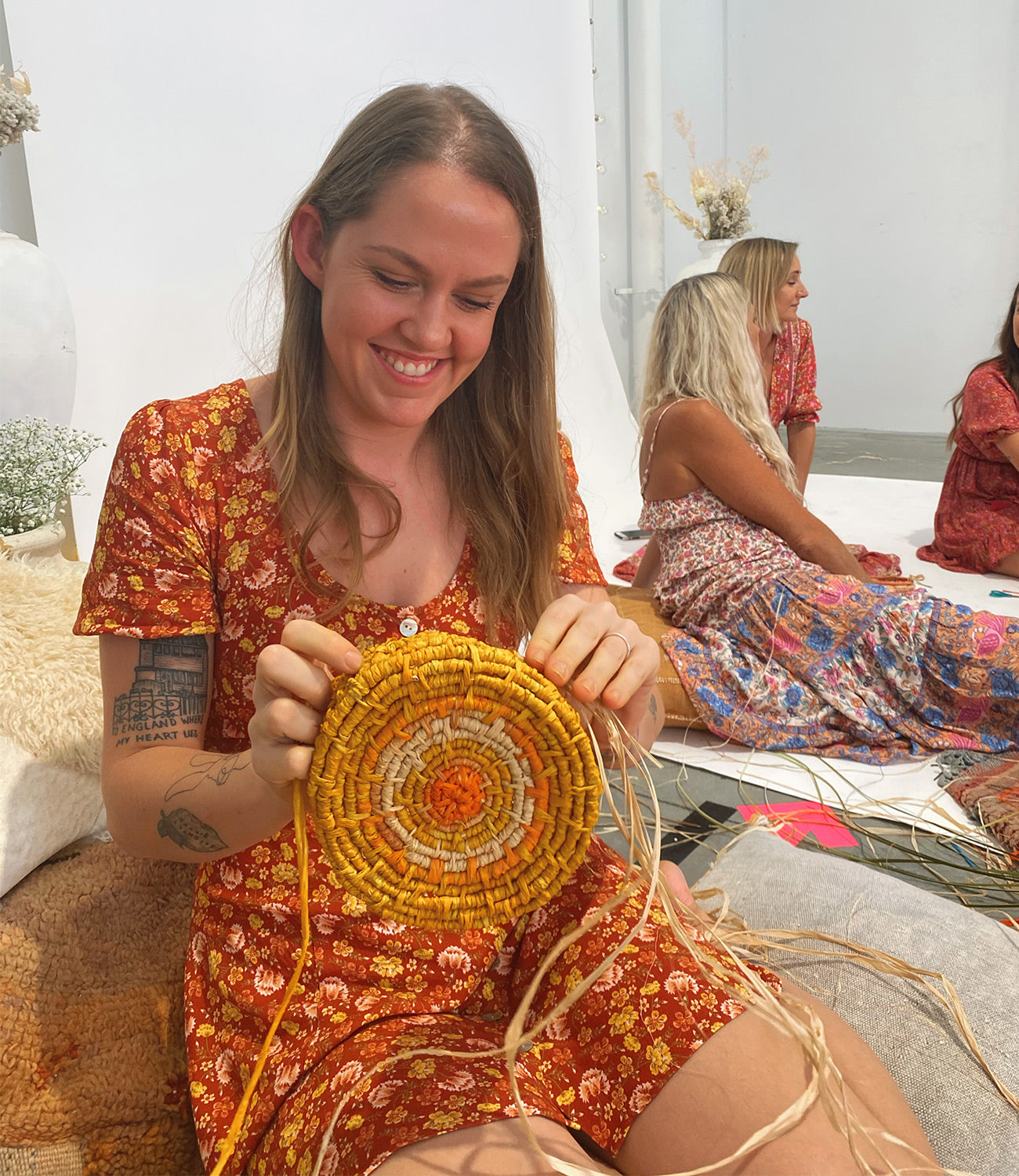In this square photograph, a young woman sits slightly left of center, facing towards the camera and smiling broadly, revealing her teeth. She has long, straight light brown hair cascading past her shoulders and wears a short-sleeved dress with a vibrant orange, yellow, and brown pattern that stops above her knees. A large tattoo adorns her right upper arm, extending down to her forearm. She is engrossed in crafting a circular wicker basket, resting on her knees and displaying an intricate design with orange at the center surrounded by layers of tan, brown, and yellow; loose pieces of straw hang from the wickerwork. The woman appears to be seated on either a chair or a collection of pillows or mats. 

Behind her, to the right, are at least three other women dressed in equally colorful, patterned sundresses. They are sitting on a sheet covering the floor and are at various angles, mostly facing away or to the right. In the background, the room features white walls adorned with plants, including a hanging plant and another potted plant on a table. The scene captures a lively and creative moment shared among these women.